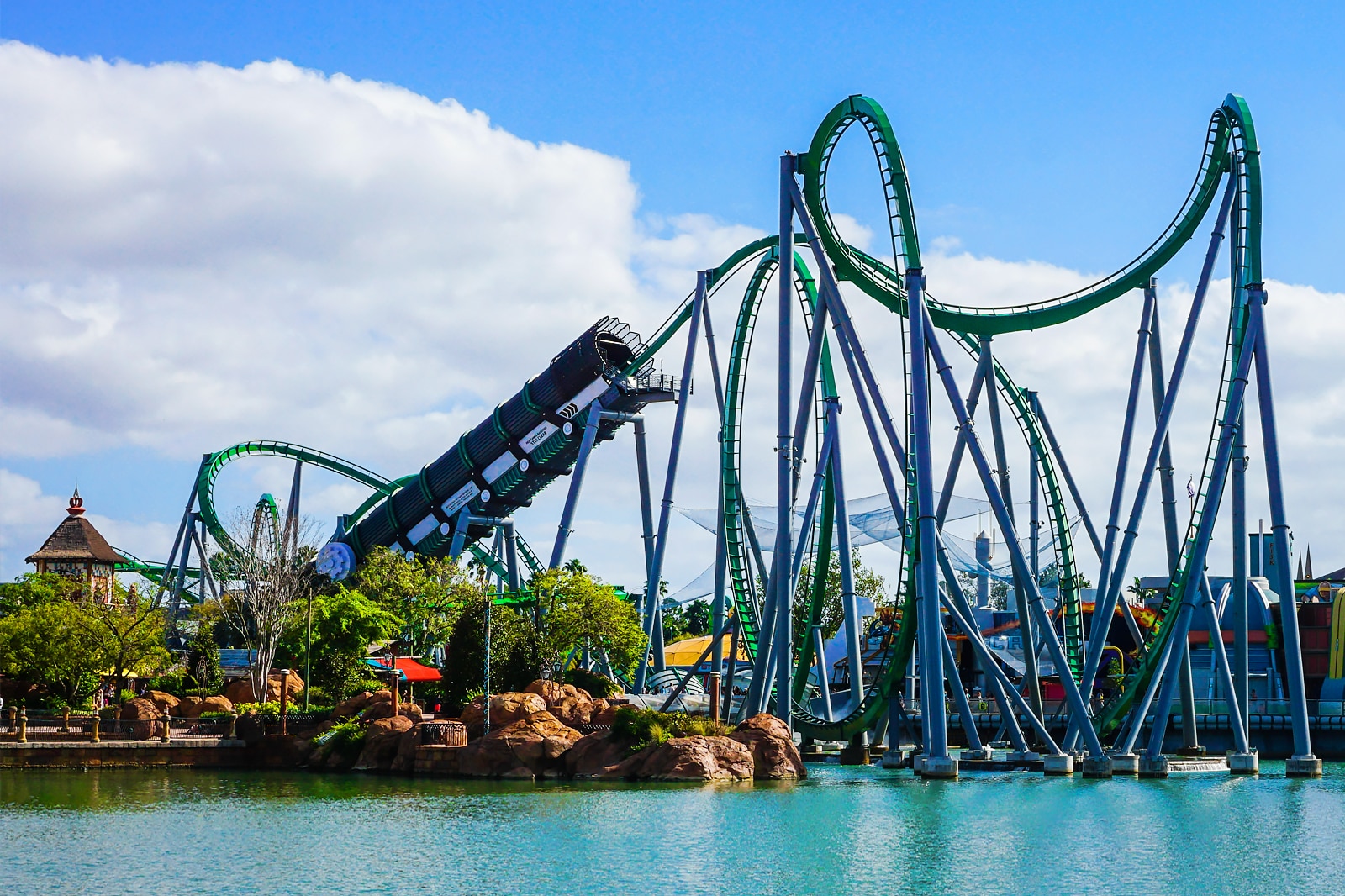This is a detailed photo of a large, green and blue roller coaster at an amusement park that also features a water park. The roller coaster, with its blue base and green upper structures, dominates the scene as it advances upwards, looping and dipping dramatically. A large green tunnel is evident at the beginning, likely where cars are shot out from. The ride extends over a body of clear, teal-colored water, whose stillness reflects the structure above. Surrounding the water are realistic-looking rocks, along with lush greenery and numerous trees.

The bottom of the image captures the serene water, transitioning into the park with stone elements and additional greenery. Buildings with various colored roofs—orange, blue, and yellow—peek in the background, hinting at other attractions within the park. Heavy white clouds dot the bright blue sky, enhancing the vibrant atmosphere. While no people are visible, nets are attached to the roller coaster, likely as safety measures. The overall scene is dynamic and colorful, encapsulating the thrilling essence of the amusement park.